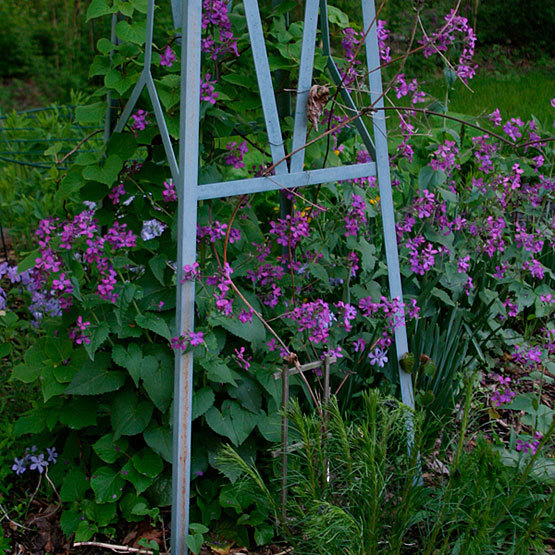The image depicts a serene garden scene centered around a vibrant flower bush adorned with delicate, light purple flowers. The lush green leaves of the bush extend from the bottom to the top of the photo, blending into the green foliage and grassy areas surrounding it. In the middle of the bush stands a noticeable wooden frame, blue in color, designed to support and guide the growth of the flowers. The frame, resembling an easel, has two visible legs at the base and forms a makeshift tower at the top. Additional garden details include patches of grass, ferns, and some weeds in the background. The overall composition captures the natural beauty and tidy organization of the garden area.